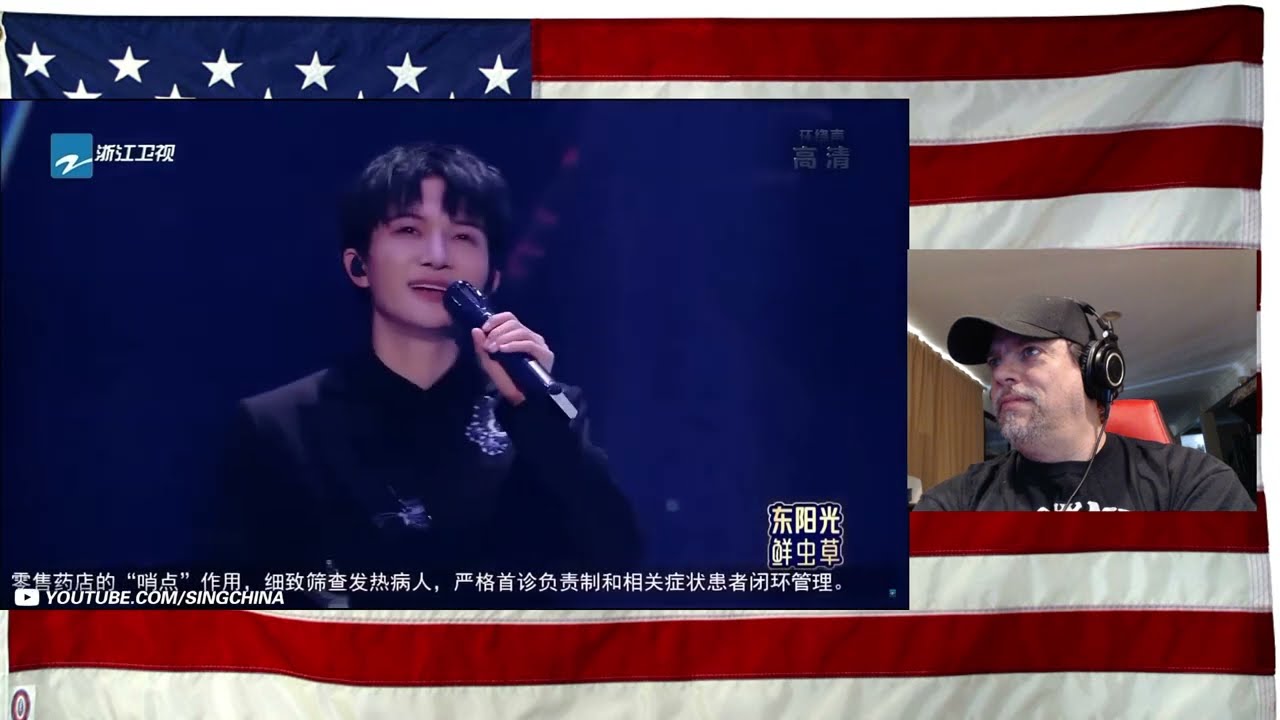The image captures a composite scene featuring elements of both a webcast and a performance. Dominating the background is an American flag, with its familiar blue field of stars and red and white stripes. Superimposed over the flag, on the left side, is a stage image of an Asian performer with short black hair and dark eyes, clad in a black long-sleeve jacket adorned with floral designs. The performer, who appears to be singing into a microphone, is framed by a blue background and accompanied by text in Oriental script, a YouTube logo, and the link "youtube.com/singchina."

To the right of the central image is a smaller inset showing a man wearing a black baseball cap, a black long-sleeve t-shirt with white writing, and a headset. This man has a white goatee and is seated on a red chair, possibly in a casual setting like a basement. He appears to be looking off to his right, which aligns with the viewer’s left, creating a sense of interaction as if he is observing the performer. The overall montage suggests a blend of American and Chinese cultural elements, curated within the framework of an online broadcast or webcast.